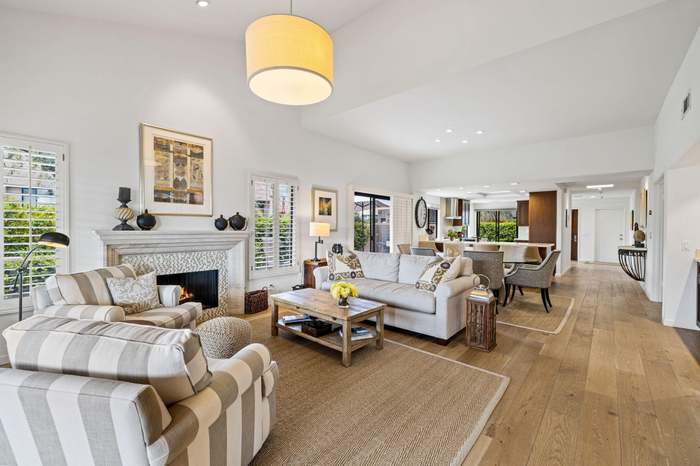This image captures a spacious and modern family room that seamlessly transitions into a kitchen area. Dominating the top of the image is a covered lamp hanging from the ceiling, illuminating the scene below. The interior design showcases a mix of contemporary and cozy elements, with two prominent white and gray vertically striped lounging chairs situated on a thin rug, which rests atop light-colored wooden floors. 

Facing these chairs is an inviting white sofa adorned with decorative throw pillows. Between the seating arrangements lies a light wood coffee table, graced with a vase of vibrant yellow flowers and other assorted items underneath. The walls and ceiling are painted white, enhancing the brightness of the room, which is accentuated by several large windows equipped with blinds that are down but open, allowing natural light to flood in.

In addition, the family room features a white fireplace adorned with a painting overhead and various decorative vases. To the side, the room expands into an elegant dining area with a table surrounded by approximately six gray chairs, continuing the airy, open-concept design. Panel doors, which are see-through, provide a view to the outside and further connect the space with the natural environment, making this interior both spacious and inviting.